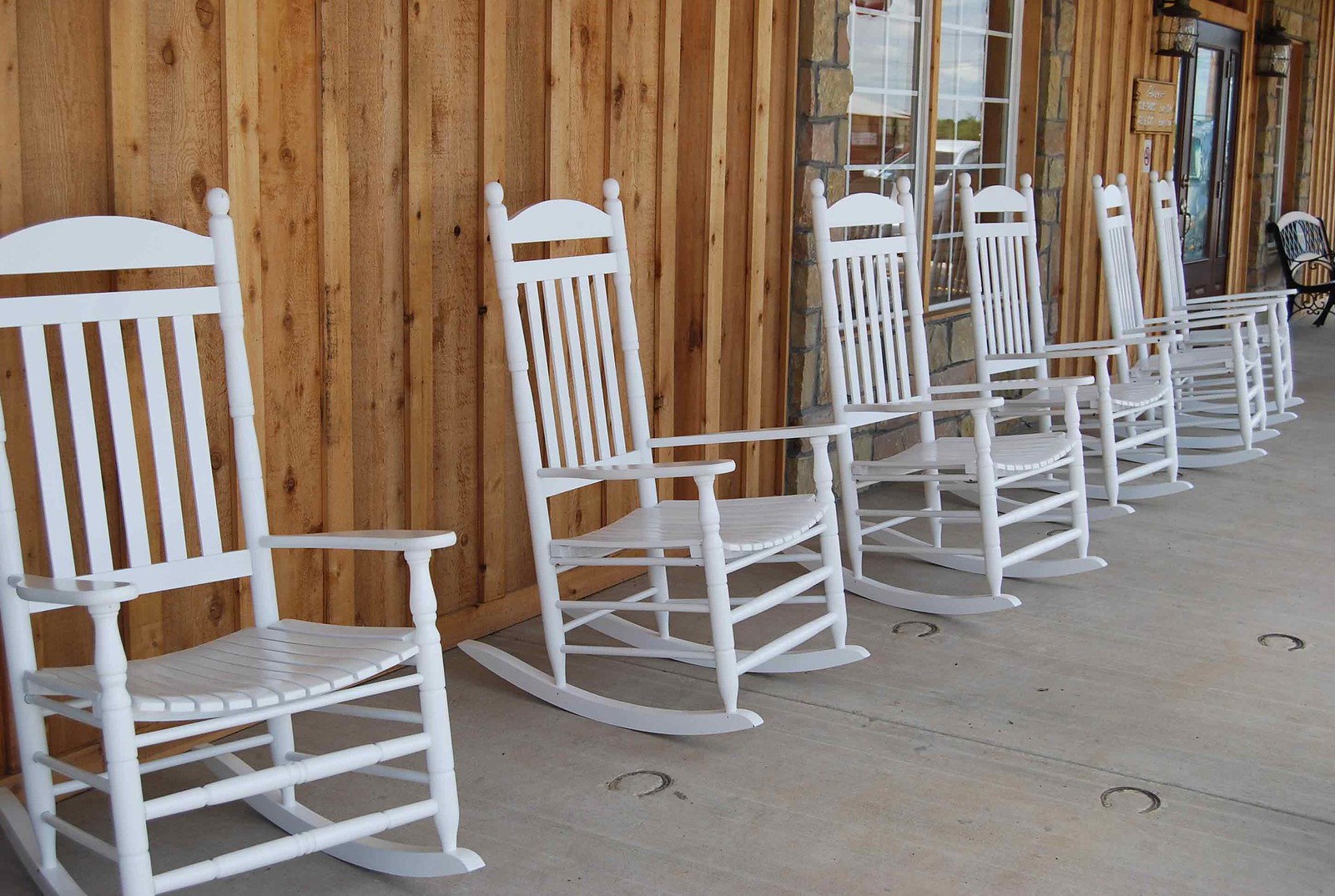The image depicts an outdoor daylight scene of what appears to be a wooden porch, possibly in front of a house or a business like a Cracker Barrel restaurant. The porch features a natural, unpainted wood exterior, with visible knots and wood grain, giving it a rustic charm. A row of six identical white wooden rocking chairs with high backs, armrests, and wood slats for seats and backs are neatly lined up in front of the house. These chairs are placed on a long concrete porch that intriguingly includes horseshoe-shaped grooves near the center. The backdrop consists of a wooden wall with vertical slats, a central window, and on the far right, a wooden door with a glass window and a bench beside it. Above the door, two porch lights flank either side, enhancing the welcoming ambiance of the porch area.